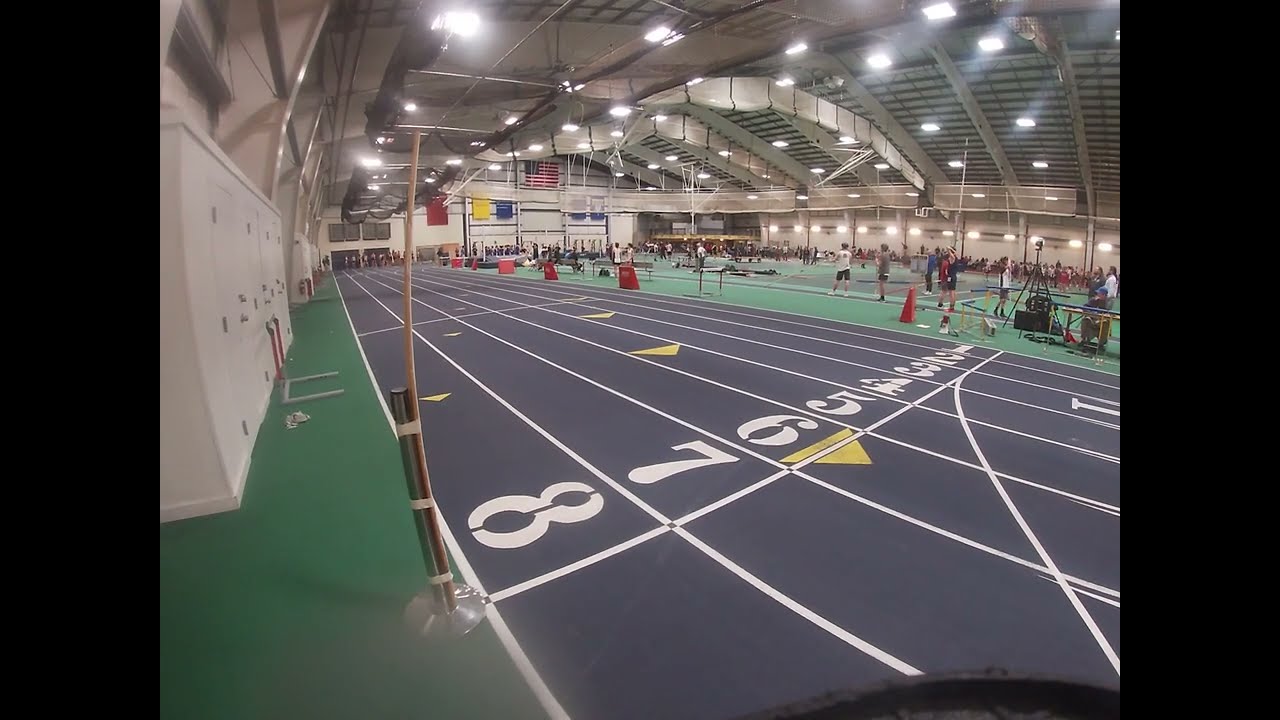The photograph captures a bustling indoor track meet held in a vast, dome-shaped arena. Dominating the foreground are the eight numbered lanes of the track, which are black with white lines – the numbers, one through eight, are clearly marked, though lane one is slightly out of focus due to the angle. The green-carpeted area in the center is populated with various figures including coaches, athletes, and officials, highlighted against the backdrop by the bright, fluorescent lighting illuminating the entire arena.

The track is left flanked by a row of beige lockers, presumably for athletes’ gear, and an American flag is prominently displayed on the far wall, accompanied by various colored banners—red, blue, and yellow—that likely celebrate the institution’s track achievements. The ceilings, composed of brown beams arching across the arena, underscore the dome's vastness, also accentuated by the sloped, white walls.

Though the track is busy with activity, no race is currently in progress. The participants are gathered mostly at the distant end of the track and within the green central area. Orange cones and other track equipment are scattered around, adding to the structured chaos of the event. The lack of visible spectator seating suggests that onlookers might be standing out of the frame or perhaps on the far side of the arena. In summary, the image portrays the energetic pause of an indoor track meet set within a well-lit, expansive, and organized environment.